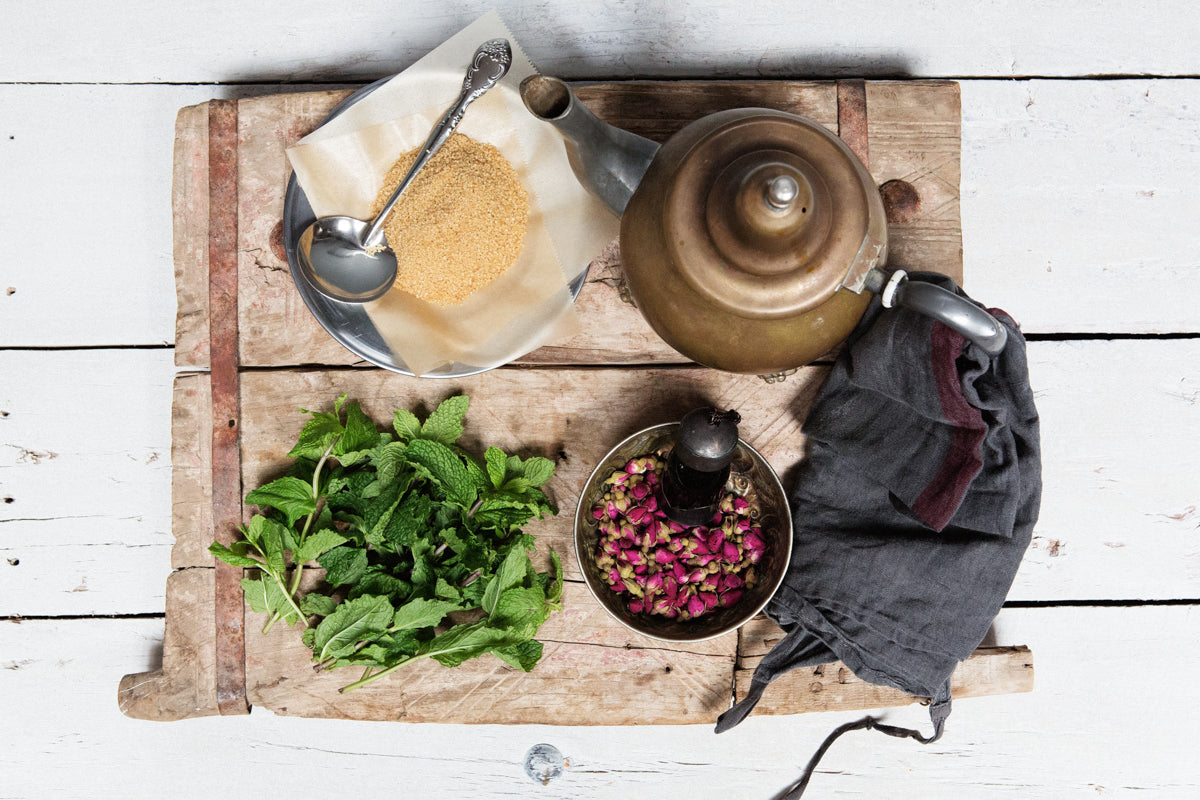In this overhead image, a rustic scene is depicted with a distressed wooden tray atop a blue-painted wooden bench. The bench features prominent horizontal slats, including a partial slat at the top, a full slat in the middle, and two-thirds of a slat at the bottom. On the tray, composed of a brown wood with darker brown stripes, various tea-making components are artfully arranged. Dominating the tray, a large piece of brown wood occupies about two-thirds of its surface. 

In the top left corner of the tray, a silver bowl contains a white cloth, holding what appears to be white grains. Diagonally across from the bowl, a large silver spoon rests, its handle extending toward the top right. Adjacent to this, a slightly rusty brown teapot with a silver spout and handle is prominently placed; a dirty blue rag is wrapped around the bottom of the handle for grip.

Toward the bottom right of the tray, a bundle of fresh mint leaves is piled together, enhancing the scene with greenery. Beside the mint, a silver container holds what looks like a mix of purple flowers and brown bits, with a small black tube-like object protruding from its rim, difficult to precisely identify. Below this container, there is what seems to be another bowl, possibly containing more herbs or ground substances, adding to the rustic charm.

Overall, the scene is one of organized disarray, creating a cozy, old-world aesthetic centered around the art of tea preparation.